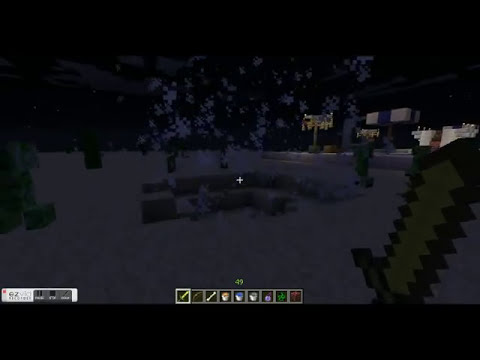The image appears to be a screenshot from the 3D video game Minecraft, displaying a pixelated, blocky environment characteristic of the game. The scene is notably dark, suggesting it is set at nighttime, making details harder to discern. The player's point of view shows them holding a yellow, pixelated sword in the lower right-hand corner. At the bottom of the screen, there is a row of item slots or options, commonly seen in Minecraft's user interface.

The environment includes a sandy area with a small pit in front of the viewer. On the left side, there are blocks or boxes stacked up, possibly part of a small fort or low walls. The right side of the image reveals a series of snowflakes falling, indicating snowy weather and white patches on the ground. Additionally, the right side shows what might be stadium lights and a blue building in the background. There is also a structure in the distance that could be a house, featuring some white and blue elements, possibly white stairs. The sky is black with faint shapes, perhaps clouds or other ambiance, contributing to the murky visibility. Overall, the scene is rich with typical Minecraft visual elements, albeit obscured by the nighttime setting.